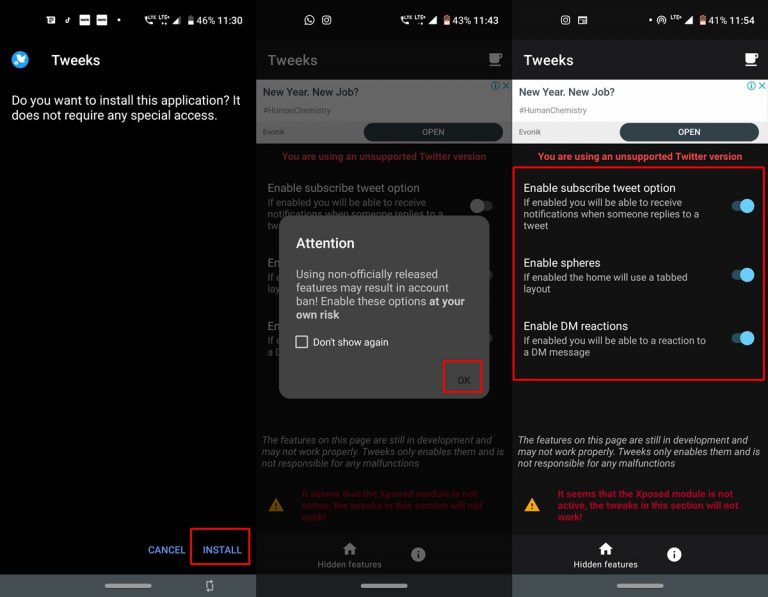The image consists of a warning screen for an application called "Tweaks" on a mobile device with a predominantly black background. The prompt asks, "Do you want to install this application?" followed by a brief explanation stating that the app does not require any special access. 

Highlighted in bold text is a caution message: "Attention, using non-officially released features may result in account ban. Enable these options at your own risk." Below this warning, there is a checkbox option labeled "Don't show again" accompanied by a red box surrounding the "OK" button on the left and the "Cancel" button on the right.

The screen further indicates, "You are using an unsupported Twitter version," and offers several experimental features:

1. **Subscribe Tweet Option:** When enabled, this feature provides notifications when someone replies to a tweet. The toggle switch for this option is in the 'on' position.
2. **Enable Spears:** When activated, this alters the home layout to a tabbed format. The toggle for this feature is also in the 'on' position.
3. **Enable DM Reactions:** This allows the user to react to direct message (DM) conversations, with the toggle set to 'on'.

A note at the bottom of the screen states that these features are still in development and might not function correctly. It further warns that "Tweakers only enable them and is not responsible for any malfunctions." Another message indicates that the "exposed meth fuel is not active," meaning the Tweaks in this section will not work currently.

The top of the screen displays the phone's status bar, and the bottom of the screen includes three white bars, possibly indicating navigation options. The entire interface has a mix of red, white, and gray elements set against a predominantly black background. A recurring red box marks critical interactive options and warnings throughout the display.